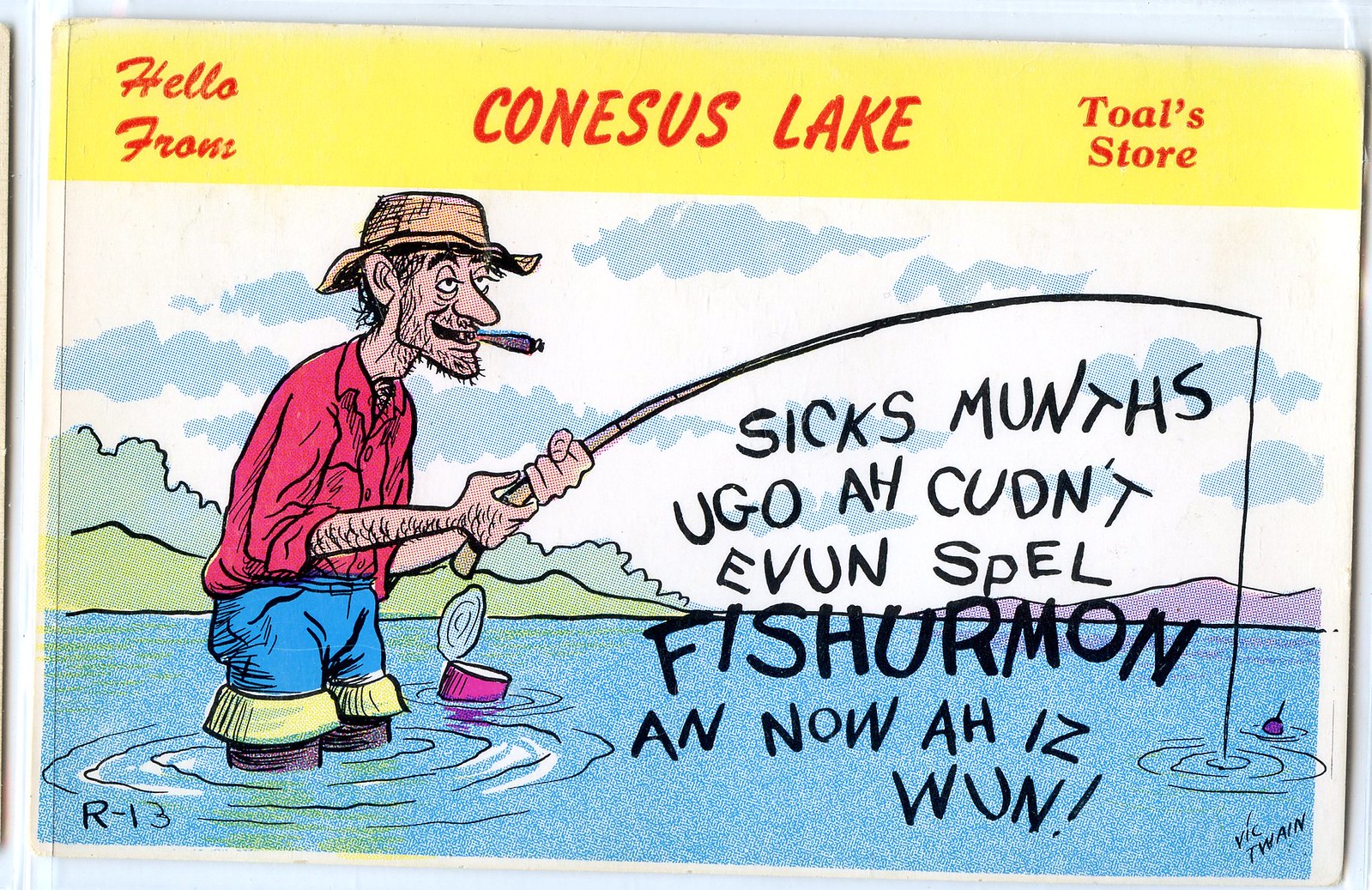The rectangular cartoon image depicts a man standing in a lake with water up to his thighs, holding a fishing rod in his hand. He is wearing a wrinkled red shirt and blue pants, along with fishing boots. An old, wrinkly hat with a brim adorns his head, and a cigar is protruding from his mouth. His face appears scruffy, as if he hasn't shaved in some time. In the background, there is a sky with scattered blue clouds and a blue mountain, all artistically drawn. The man's fishing bobber is visible in the water. 

Text in black, crooked font is positioned under his fishing rod, reading, "Six months ago ah couldn't even spell Fishermon and now ah is one," with several spelling errors. Above the entire cartoon drawing, there is a horizontal strip of yellow color featuring additional text. On the left side, it says, "Hello from," in the middle, "Connoisseurs Lake," and on the right side, "Toll's Store."